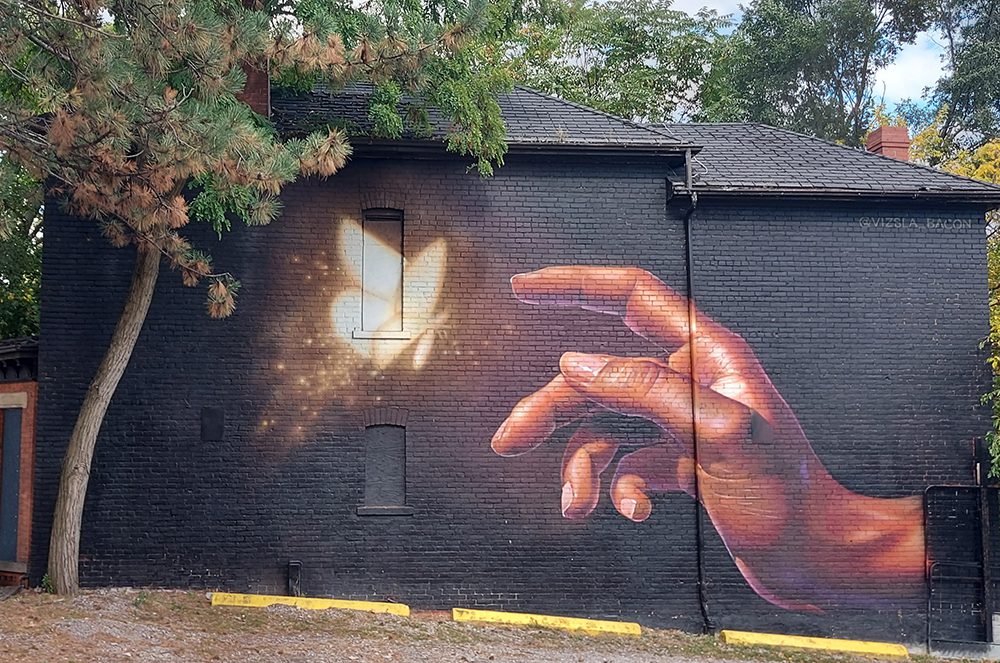This photograph captures a striking, two-story house constructed from black bricks, featuring black rooftops, and black windows. The house, likely set in a forested area, is framed by several trees, including a prominent pine tree on the left with brown and green needles, indicating a transition into fall. A red brick chimney adds a distinct contrast at the top right of the building. The side of the house serves as a canvas for an evocative urban mural: a beautifully detailed, dark-skinned hand reaches out towards a fluttering yellow butterfly with glowing yellow dots of light emanating from it. The butterfly appears to interact with one of the upper windows, creating a mesmerizing focal point. At the house's front, a gravel driveway is bordered by three yellow-painted curbs. The overall scene is both captivating and thought-provoking, blending the starkness of the black house with the vibrant and meaningful street art.